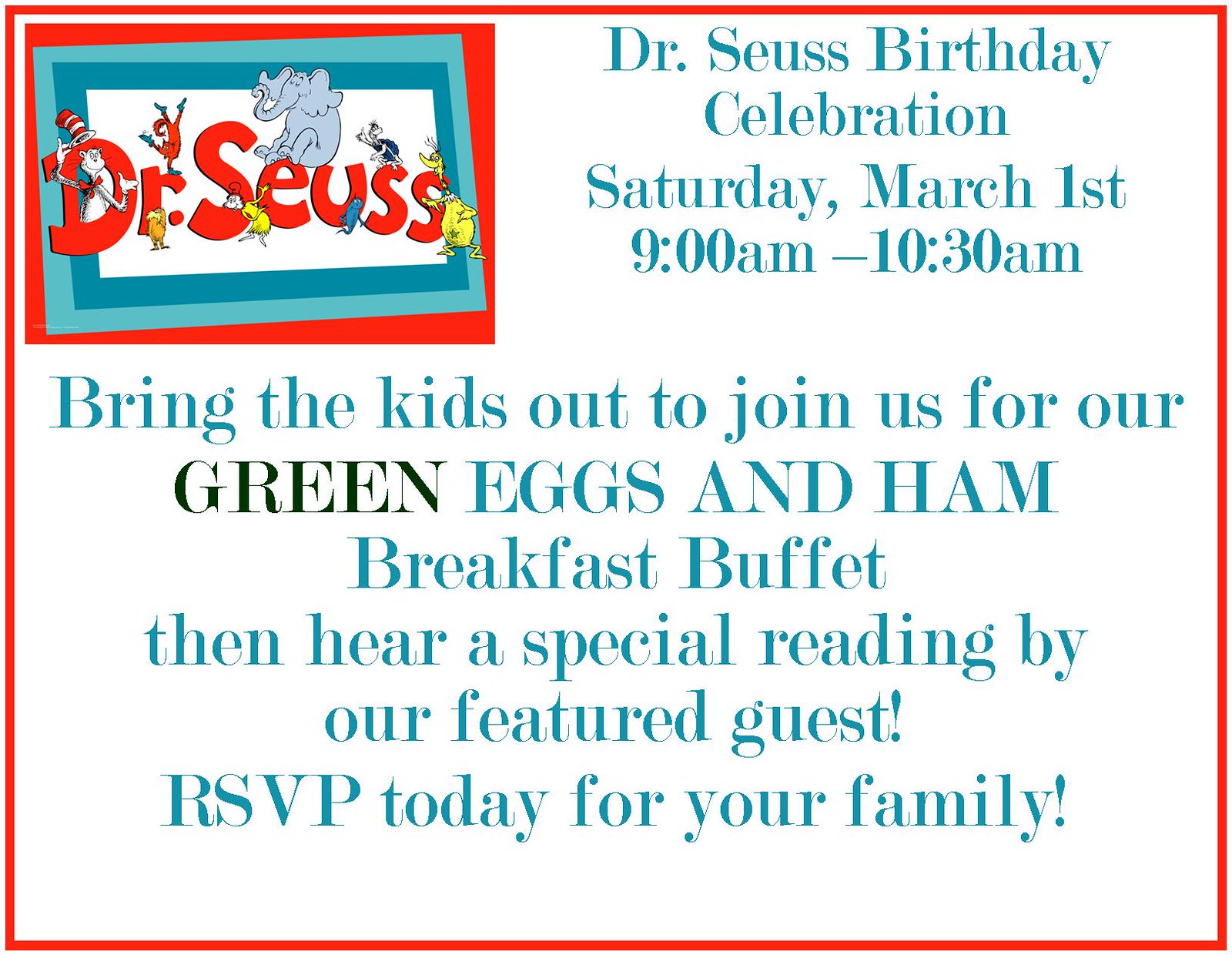This flyer features a clean, white background with a vivid red border encapsulating its entirety. In the upper left corner, a playful red square houses a smaller blue square, which in turn encases an even smaller white square—a distinctive design element framing the text "Dr. Seuss." Surrounding this logo, an array of beloved Dr. Seuss characters come to life, including the Cat in the Hat, Horton the Elephant, Thing 1 and Thing 2, and the Lorax.

In the upper right corner, bold blue text announces: "Dr. Seuss Birthday Celebration," detailing the event date as Saturday, March 1st, from 9:00 a.m. to 10:30 a.m. Beneath this, the flyer invites families to "Bring the kids out to join us for our Green Eggs and Ham breakfast buffet," with the word "Green" notably highlighted in a darker green or black font. The occasion promises a special reading by a featured guest, emphasizing the need to "RSVP today for your family." Notably absent, however, is information on how to RSVP, such as a phone number or email address.